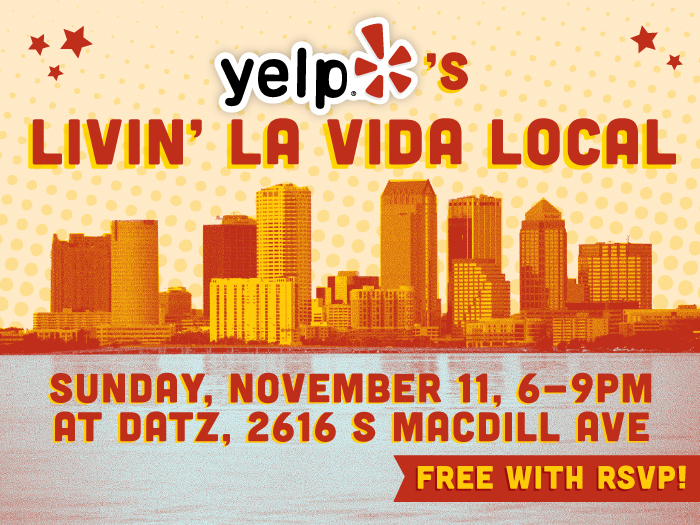This is a detailed photograph of a vibrant advertisement for Yelp. At the top, the prominent Yelp logo is displayed alongside the lively caption, "Yelp's Live in La Vida Local," or possibly, "Yelp's Live in La Vida Social." The event is scheduled for Saturday, November 11th, from 6 to 9 p.m. at Dad's, located at 2616 South MacDill Avenue. 

In the background, there is a cityscape of an unspecified major city, which does not appear as dense as New York City. The sky above the skyline features yellow polka dots on a white backdrop. A red ribbon is situated at the bottom right corner of the ad and it reads "Free with RSVP" in a gold-colored font. Additionally, the advertisement includes three red stars in the top left corner and two red stars in the top right corner. The ad itself is predominantly orange, with lettering in shades of red, dark red, and a burnt orange hue, contributing to the dynamic visual appeal.